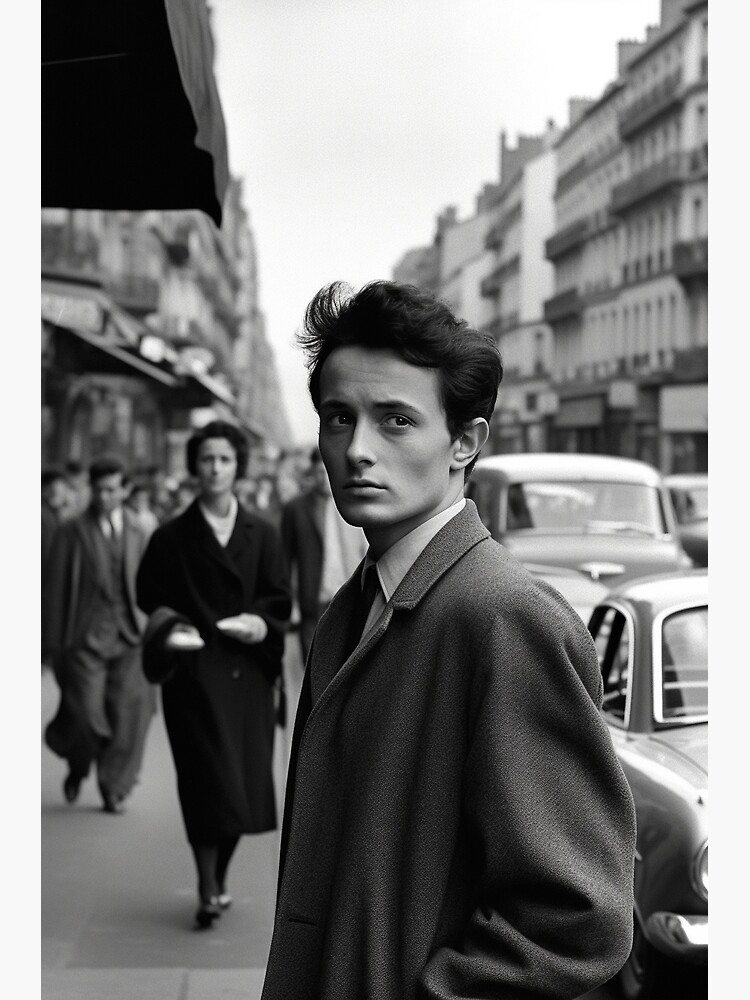The image is a sharp, retouched black and white portrait from the late 1940s or 1950s, featuring a young man prominently at its center. The man is wearing a gray trench coat over a white button-up shirt, with his hands in his pockets and his unbuttoned coat revealing a tie. He has short, black hair brushed back and is staring slightly to the right with a contemplative expression. The scene is set on a pedestrian pavement made of various gray concrete tiles, amidst a bustling cityscape. In the background, numerous people are walking, including a woman in black high heels and a long black coat with her hair pulled into a bun. To the left of the man, another woman in a long black coat is walking towards him. On the right side of the image, vintage 1950s cars are parked along a street lined with short buildings. A small black canopy extends from a shop on the top left corner of the image, adding to the vintage urban ambiance.